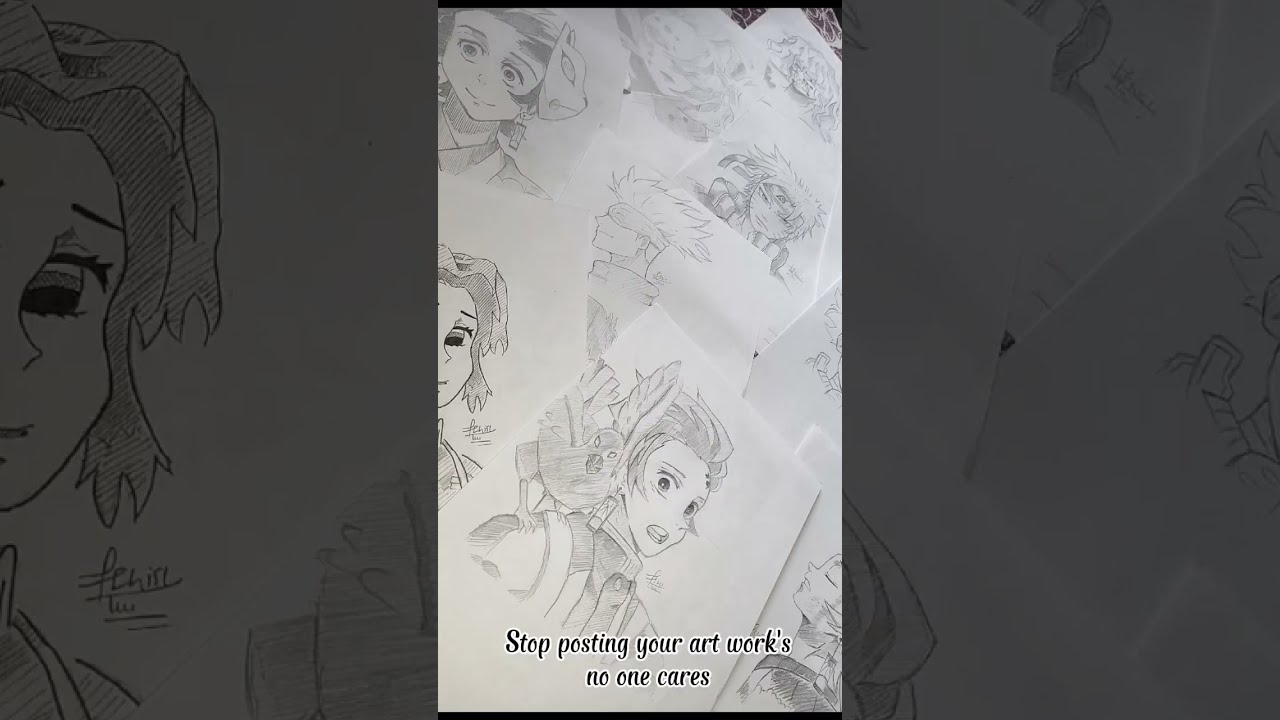The image depicts a chaotic collage of pencil-drawn anime artwork scattered over a surface. Each drawing is rendered in shades of black, white, and gray, creating a monochromatic and moody atmosphere. Central to the composition is a vivid array of pictures showcasing a variety of anime characters, including recognizable figures like Tanjiro from Demon Slayer and Gojo from Jujutsu Kaisen. The characters exhibit exaggerated anime features such as large, expressive eyes, detailed hair, and dramatic facial expressions. Among them is a girl with a shocked expression, large eyes, and a small bird perched angrily on her shoulder. Another notable figure is a male with a bandana and spiky hair, and there’s also a female character adorned with a cat mask.

Flanking the main artworks are zoomed-in, darker versions of the same drawings, adding depth but making specific details harder to discern. At the bottom center of the image, a bold text message reads, “Stop posting your artworks, no one cares,” underscoring an anti-artwork theme. This text, written in black with a contrasting white outline, serves as a stark commentary on the value and reception of art.